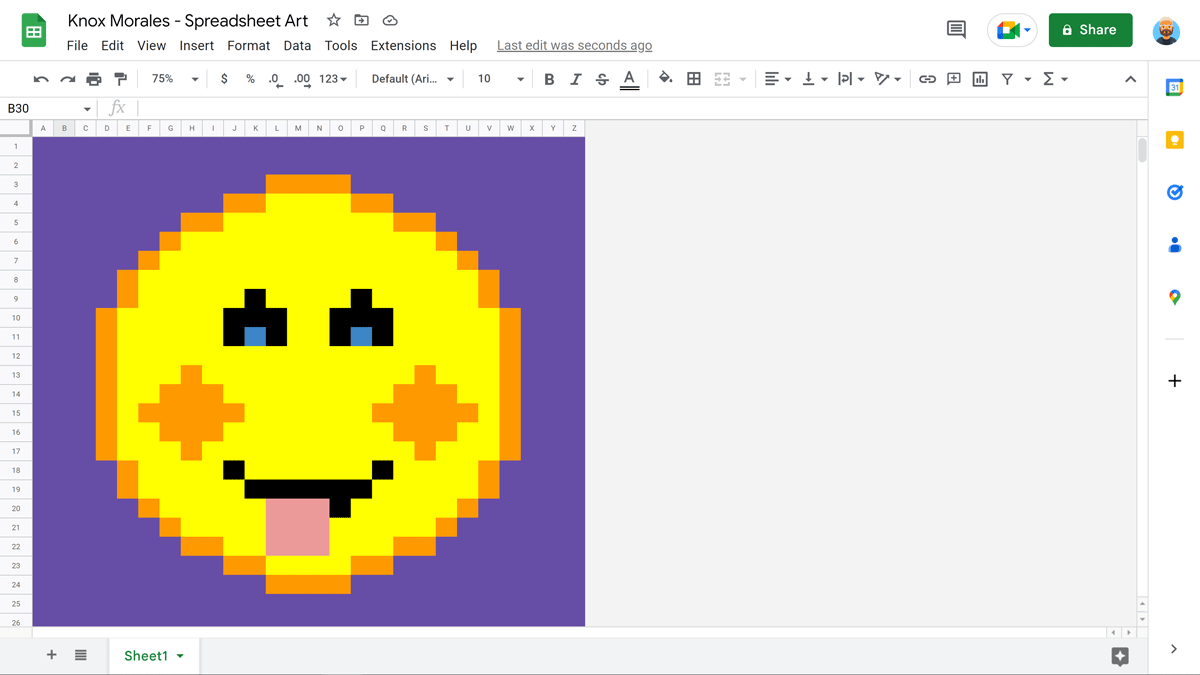The image is a screen capture of an Excel sheet transformed into a piece of pixel art titled "Knox Morales Spreadsheet Art." The pixelated drawing, formed by individual cells, features a vibrant smiley face centered on the left side of the sheet. This smiley face has a yellow circular head outlined in orange, adorned with orange cheeks, black eyes with blue centers, and a black mouth with a pink tongue playfully sticking out. The background surrounding the smiley is a solid purple, providing a stark contrast. The right side of the sheet remains plain gray. Above the artwork, the typical Excel menu bar is visible with tabs such as File, Edit, View, Insert, Format, Data, Tools, Extension, and Help, along with various tool icons for saving, printing, and text formatting options like bold, italic, and underline.